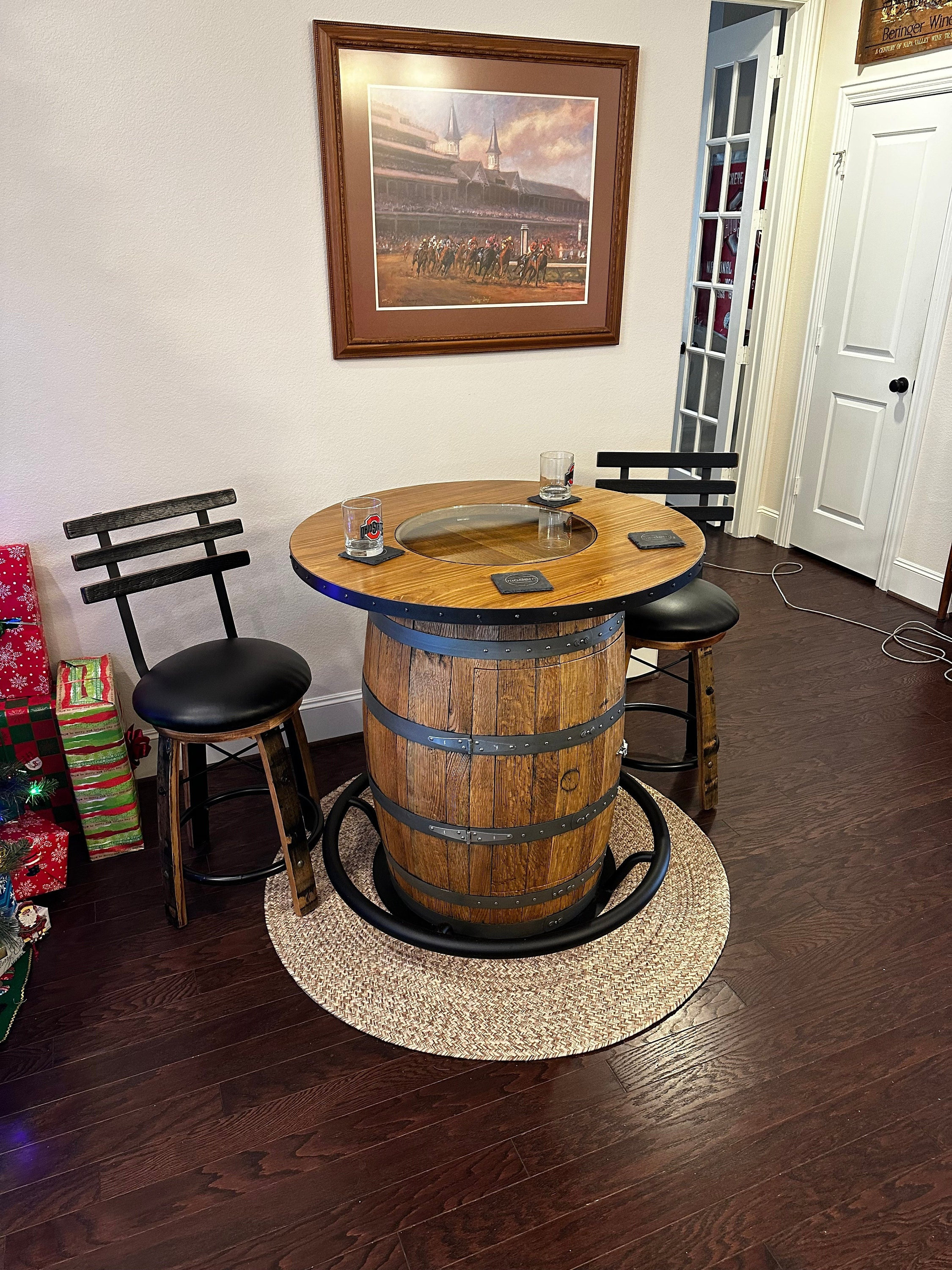This detailed image depicts a cozy room in a house, featuring a blend of festive, rustic, and modern elements. Dominating the center is a uniquely styled wine barrel table with a rich brown finish and steel trim. The barrel is converted into a table with a round wooden top, adorned with two glasses featuring Ohio State logos and black coasters. Surrounding the table are two black stools, which have black wrought iron frames and wooden legs, each with three black slats forming the backrest. The table and stools rest on a light brown round rattan rug, contrasting with the dark chocolate brown wooden floor.

On the left side of the image, brightly wrapped Christmas packages peek out beside a glimpse of a Christmas tree, adding a festive touch. The back wall, painted white, showcases a squared brown-framed picture capturing the dynamism of a horse race, complete with jockeys, horses, and a stadium in the background.

To the right, a French door with glass panels leads to another room, accompanied by a solid white door. A white cable runs along the floor, leading into another room. Above the door, there is a brown sign. Additionally, a slight hint of a yellow wall is visible, contributing an extra layer of color to the setting.